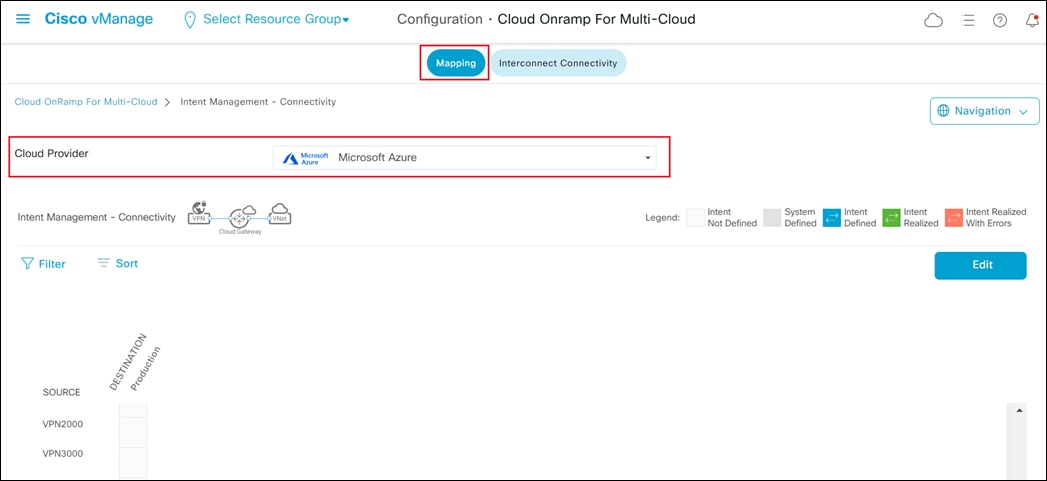This image is a screenshot taken from a computer, displaying the Cisco vManage interface. At the top of the screen, "Cisco vManage" is prominently featured in blue text. To its right, there's a pin icon accompanied by the text "Select Resource Group" and a corresponding dropdown menu. Moving further to the right along the top bar, the labels "Configuration," "Cloud onRamp for Multi-Cloud," a cloud icon, three horizontal lines, a question mark within a circle, and a bell icon with a red notification dot can be seen.

In the middle section of the interface, there's a blue button labeled "Mapping," which is highlighted with a red-drawn rectangle around it. Beside this, there is an "Interconnect Connectivity" button. As the view progresses downward, the section titled "Cloud onRamp for Multi-Cloud" with further sections "Internet Intent Management" and "Connectivity" is visible. Below "Connectivity," an area designated for cloud providers displays "Microsoft Azure," which has also been highlighted with a red rectangle and border.